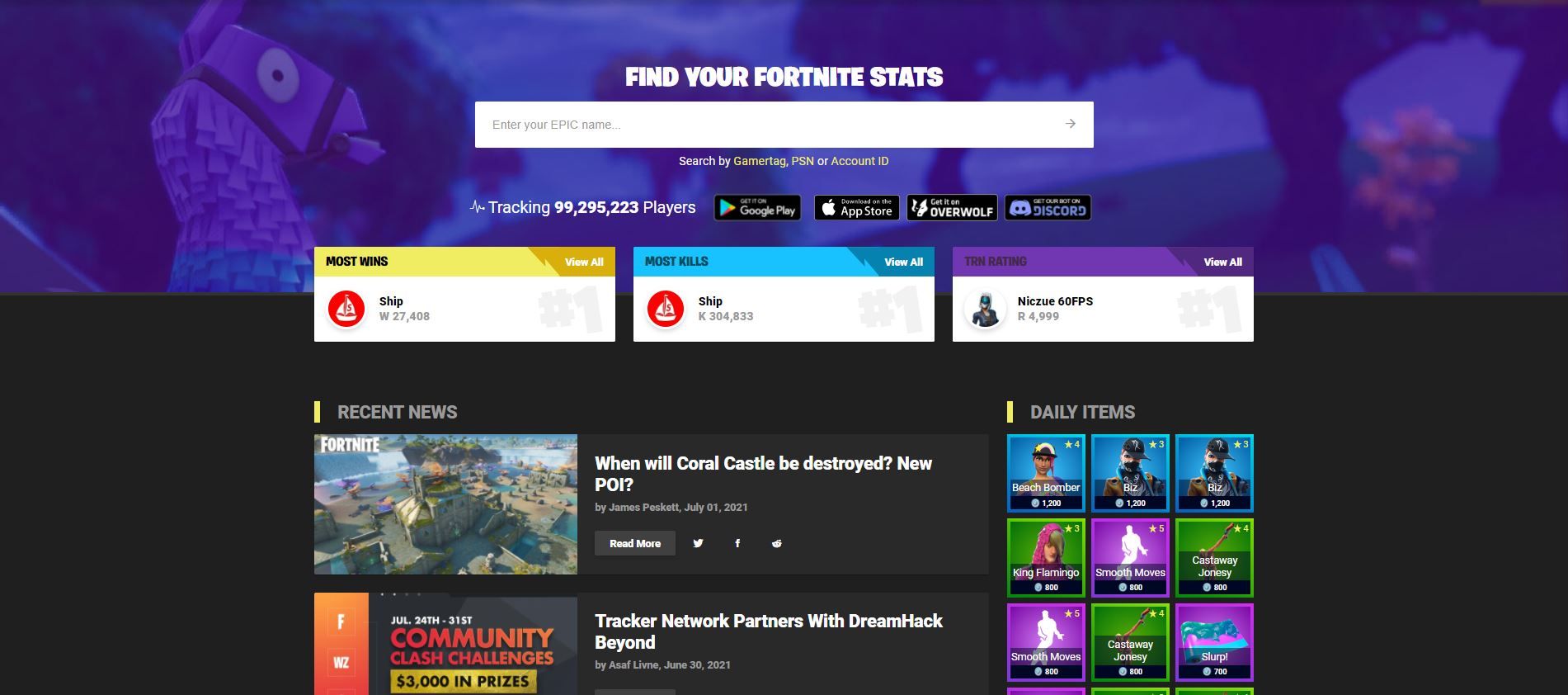Screenshot from Fortnite Stats Page

The screenshot showcases a visually appealing page from the game Fortnite, characterized by its vibrant and dynamic elements. Dominating the top third of the screen is a captivating purple section, possibly portraying a futuristic, robotic horse with intricate design. The purple area features ethereal purple smoke and small windows revealing a serene blue sky.

Below this striking header are three boxes in different colors: yellow, blue, and purple. Each section seems to serve a specific function or category. Further down, the page is divided into two main sections: "Recent News" on the left and "Daily News" on the right. 

The "Daily News" segment, though somewhat unclear, displays images depicting people engaged in various activities. Notably, one image appears to show a tanker. Beneath this section, there is mention of the community and a banner highlighting $3,000 in prizes. 

Overall, the page combines engaging visual elements with practical information, appealing to both new and seasoned Fortnite players.